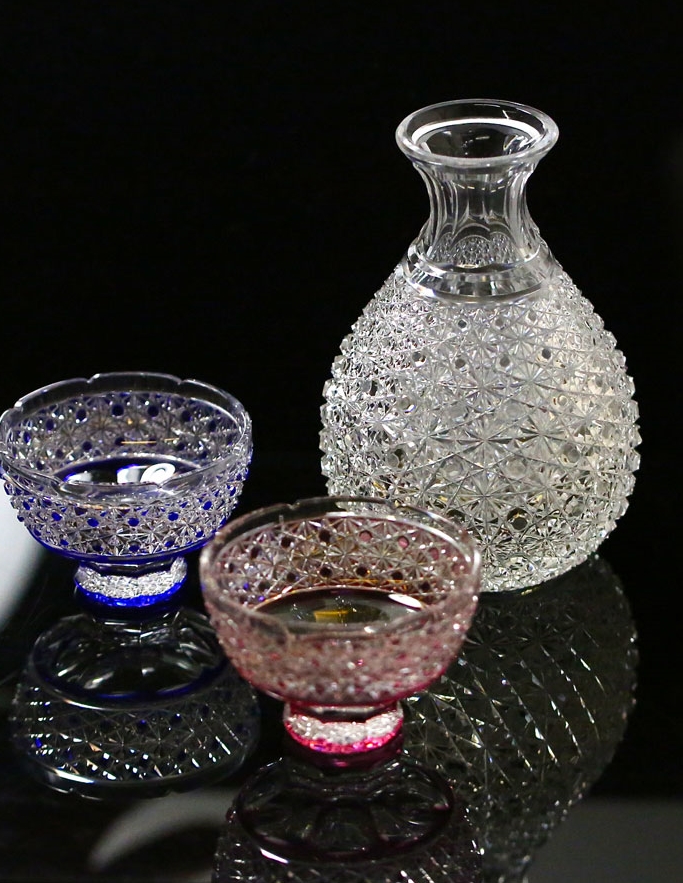This image features three intricately designed crystal vases displayed against a pitch-black background on a glossy, black-tinted reflective surface. The vase on the right is the largest, with a clear crystal body and an ornate geometric pattern composed of numerous intricate triangular designs. It has a wide, circular base that tapers into a narrow neck, ending in an open spout at the top.

To the left are two smaller, bowl-shaped vases. The one further from the center is predominantly blue with scattered blue dots and a matching rim, also adorned with similar geometric designs as the larger vase. Closer to the center, the second smaller vase has a pink tint with a pink-hued base and rim, showcasing the same detailed line patterns present in the other pieces. Each vase casts a vivid reflection on the smooth, black surface, adding depth to the composition and highlighting the precise craftsmanship of the crystal and its decorative elements.